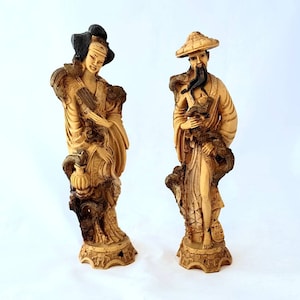The image features two porcelain figurines, set against a blue background, representing Asian characters. On the left stands a woman with thick black hair styled into three distinct buns. She is attired in a flowing kimono-like dress adorned with brown highlights and is holding her kimono closed with her left hand. By her side, there's an ivory-colored vase with something black emerging from it. She stands atop a pedestal, distinguished by half-oval cutouts. To the right is a man wearing a triangular-shaped hat and a traditional long black beard that appears to be sectioned into three braids. Clad in robes, he holds a dark brown object with both hands at his chest, with his right hand positioned above his left. One of his legs protrudes from his clothing, showing something black around his ankle. He is also positioned on a similar pedestal featuring three half-oval cutouts. Both figurines exhibit a detailed and intricate design, reflecting Asian craftsmanship.